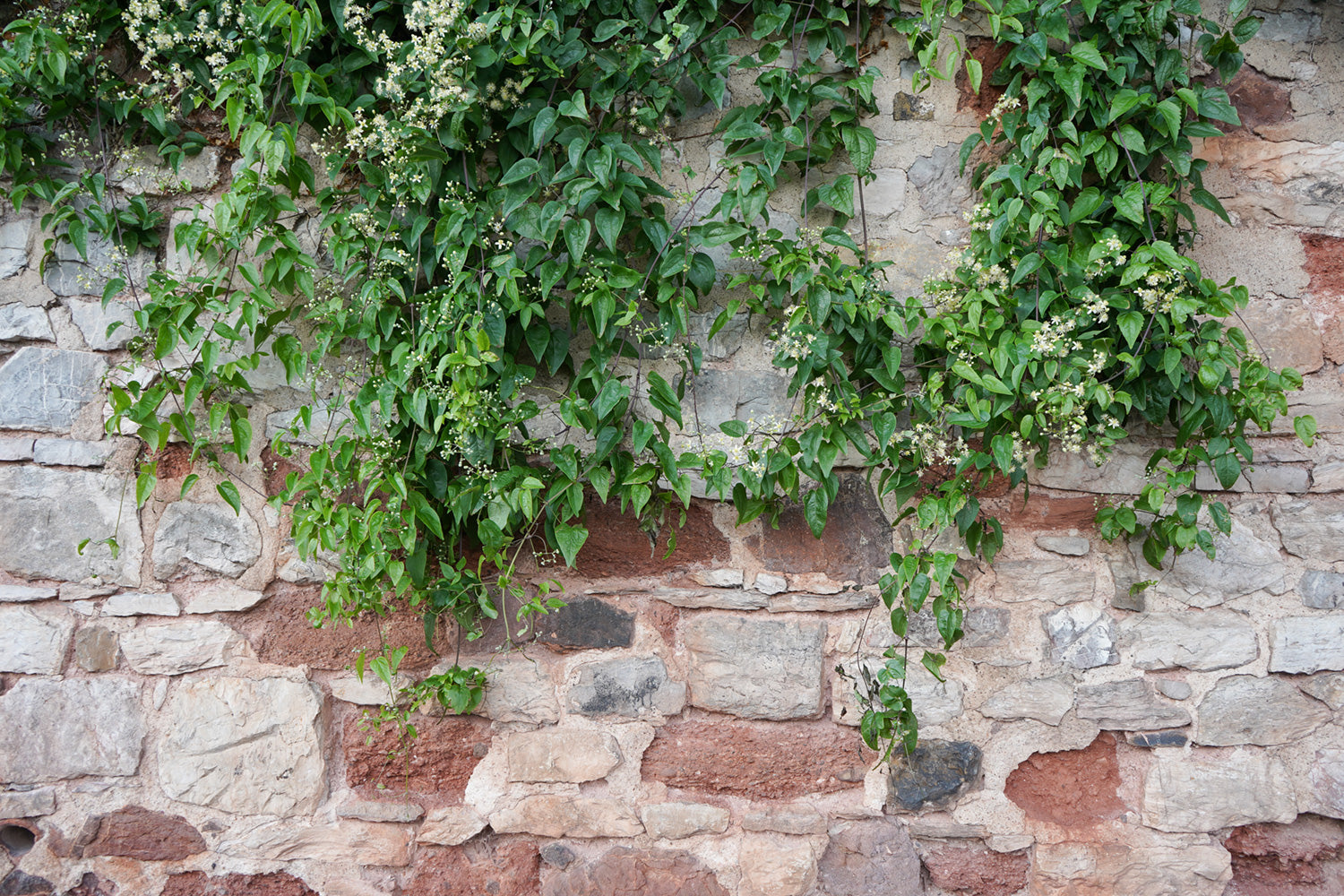The image captures a close-up, daylight shot of a man-made stone wall, showcasing its varying shades of grayish-white stones interspersed with reddish-brown and darker gray rocks, particularly prominent near the bottom. Flanking the top of the wall are lush, green, leafy vines adorned with delicate white flowers. These vines cascade down, extending past the midpoint of the image but not quite reaching the bottom, creating a natural curtain. The overall composition suggests an outdoor setting, possibly in a courtyard, emphasizing the vibrant contrast between the structured stonework and the organic flow of the flowering vines.